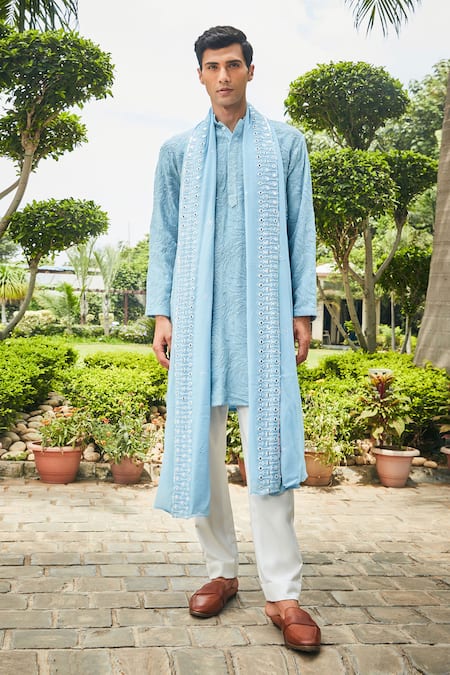The image features a male model, an Indian man with short dark hair, standing in an outdoor garden setting. He is dressed in a light blue embroidered kurta with long sleeves and buttons, which extends to about mid-thigh. Complementing his attire is a matching light blue scarf draped over his shoulders, with both ends extending past his knees and adorned with white embroidery. He pairs the kurta with white pants and brown leather slide sandals. The model stands on a walkway made of brick pavers. Behind him, the garden boasts terracotta planters filled with various green plants, river rocks, lush green shrubs, and tall, slender trees with bushy green tops. The sky above is white and cloudy, adding to the serene ambiance. The man gazes directly at the camera, adding a composed and engaged presence to the scene.